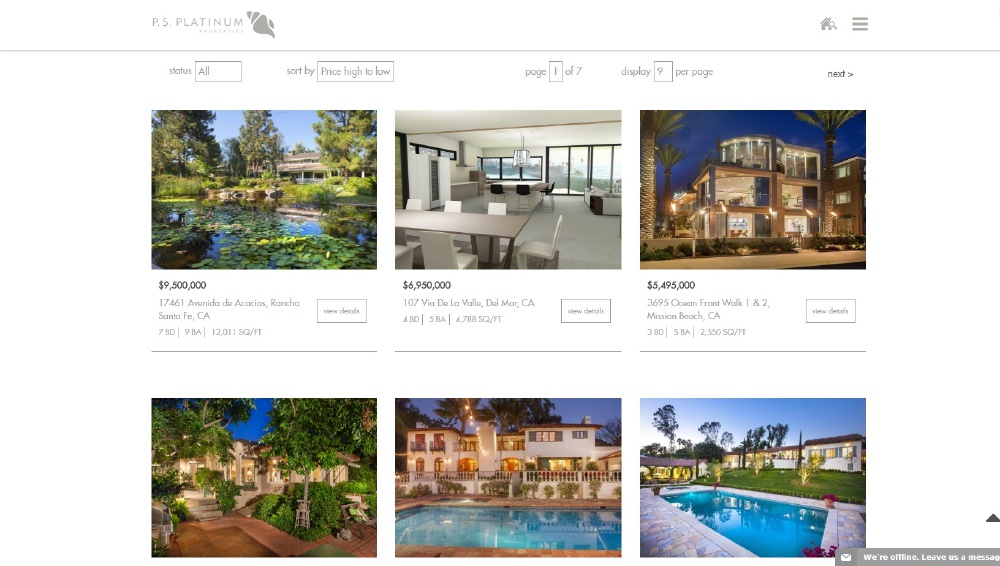This image is a screenshot of the website "PS Platinum," identifiable by a light gray title and a seashell-shaped logo located in the top left corner. The central section of the webpage prominently displays six luxurious properties, each represented by a large photograph. These properties are expansive multi-story homes, each with price tags in the millions, including $9 million, $6 million, and $5 million listings. Notable features in the images include large backyard pools and lush, tree-filled surroundings. One property also showcases a detailed view of its interior, while the other five are pictured from the outside. The website has a clean white background and paginates listings, displaying nine homes per page. The screenshot reveals the user is currently on the first page, viewing properties sorted from highest to lowest price.